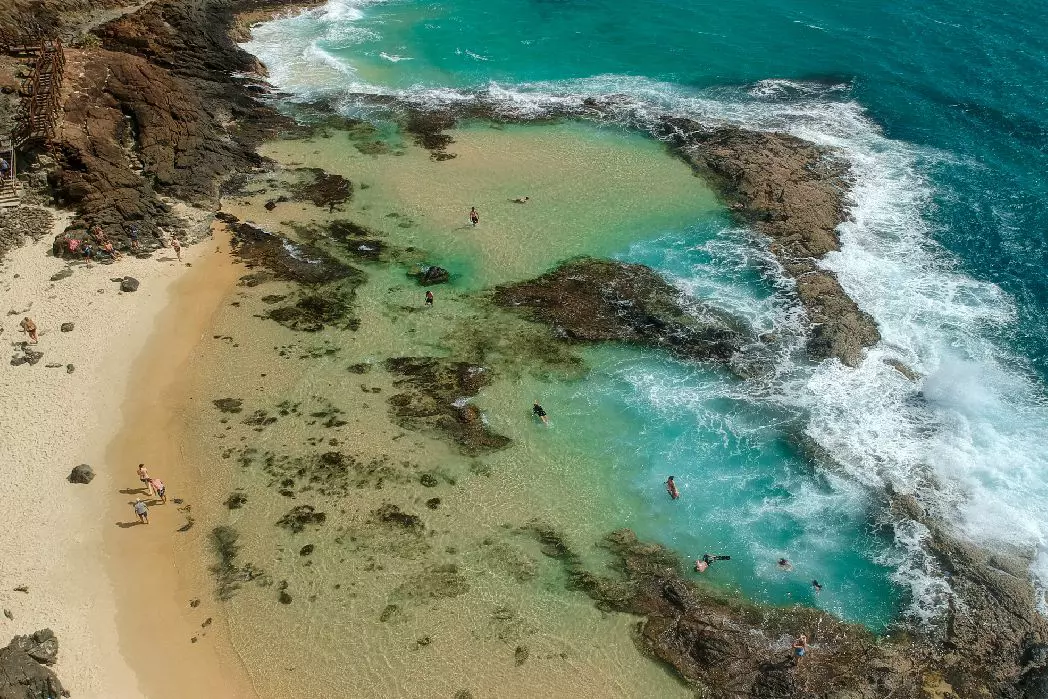This is a zoomed-out aerial photograph of a unique beach where the land meets the water. The image captures a serene coastal scene, marked by a variety of natural structures including brown cliffs and rocky embankments. These rocky formations shelter two smaller wading pools, keeping their waters calm for the numerous people swimming within them. The beach itself is honey-colored, with visitors standing along the shoreline and even sitting alongside the rocks.

In the upper left-hand corner of the image, a stairway is visible, implying that visitors likely reached the pools via this path. The water exhibits a range of colors: beginning with a clear, turquoise hue nearest the shore, it transitions to deep blue as it extends outward, while white waves crash against the larger rocks. The beach and wading pools are bustling with activity, populated by groups of people enjoying the tranquil yet dynamic interaction of sand, rock, and sea.